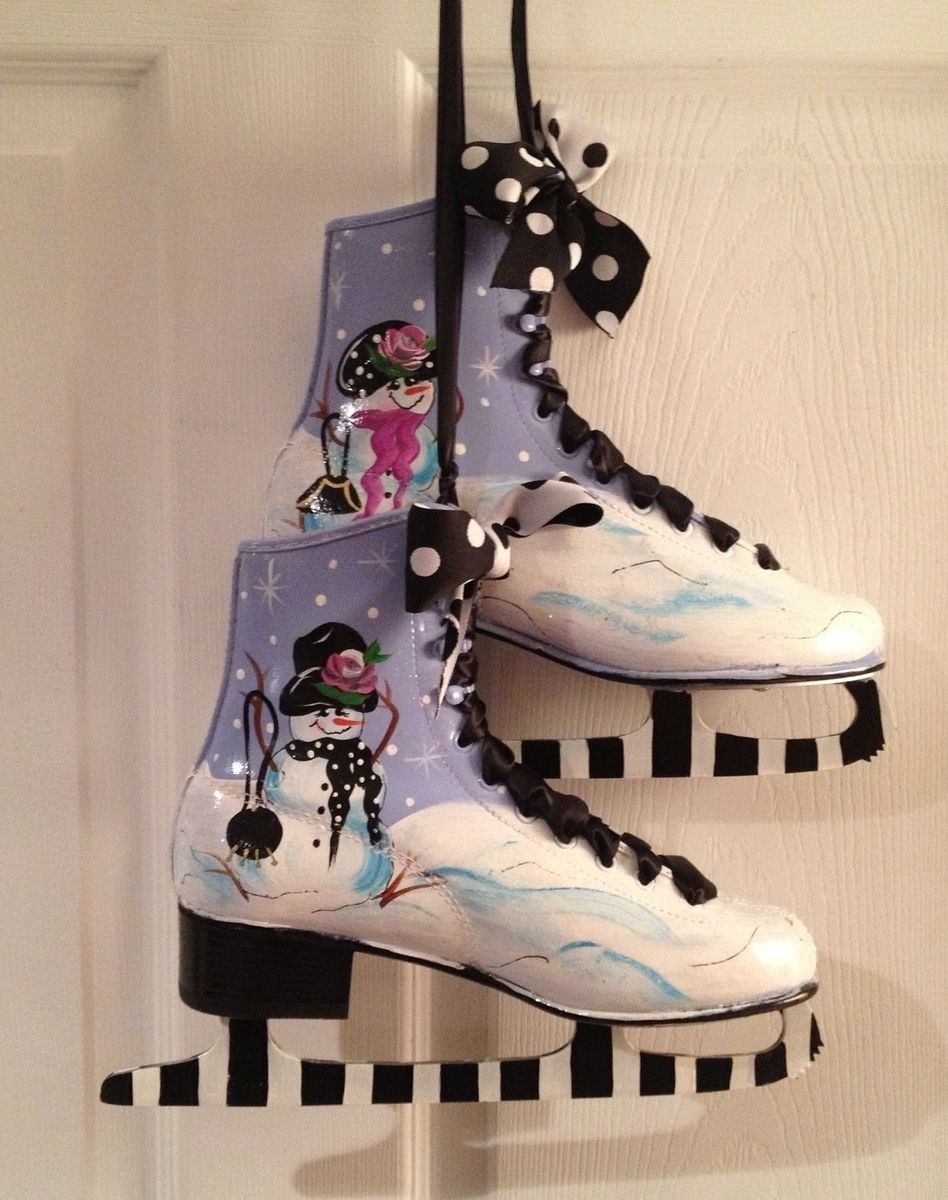This photograph showcases a whimsical pair of ice skates ornately decorated and hanging from the top of a white wooden door. The skates feature custom-painted designs, with the blades adorned in black and white stripes. The boots of the skates are painted in vibrant purple and depict a charming female snowman positioned by the heel. The snowman holds a tiny black purse with her branch-like arms raised joyfully. She sports a black and white polka dot scarf, a broad smile, and wears a large black hat adorned with a pink rose. The background surrounding the snowman is a snowy landscape that extends down to the toes of the skates. Completing the festive look, the skates are laced with black and white polka dot ribbons, tied into delicate bows at the top.